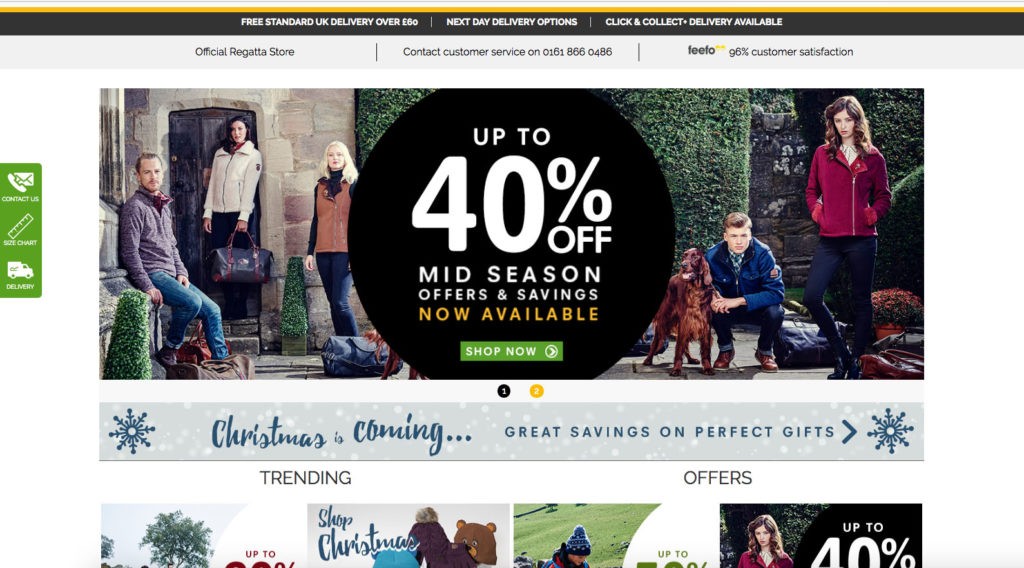**Detailed Caption:**

This image is a screenshot of a business's web page. At the very top, there is a prominent black bar spanning the full width of the page, displaying essential shipping information: "Free standard UK delivery on orders over £60," "Next day delivery options," and "Click and collect delivery available."

Below this, a gray navigation bar is visible, highlighting key service points such as "Official Regatta Store," "Contact Customer Service," and "FEEFO 96% Customer Satisfaction."

The main section of the webpage features a vibrant image of a group of well-dressed individuals, showcasing high-end attire. Centrally placed over this image is a striking black circle with white text that announces "Up to 40% Off, Mid-Season Offers and Savings." The circle is accented with a bold yellow label stating "Now Available" and a green rectangular button that prompts with "Shop Now" in white text.

Underneath the central image, there is a festive banner proclaiming "Christmas is coming, great savings on the perfect gifts." This banner has a subtle gray background adorned with softly falling white snowflakes. At each end of the banner, there are blue snowflake graphics, further enhancing the holiday theme.

Following the festive promo, the webpage features a heading labeled "Trending." Partially visible under this heading is an image of a tree alongside another image labeled "Shop Christmas." Adjacent to this section, another heading reads "Offers," featuring visuals of someone wearing a hat on the grass and another well-dressed individual, with a clear mention of "Up to 40% Off" discounts.

This detailed overview captures the essence and structure of the web page, ensuring that all key visual and textual elements are highlighted clearly.